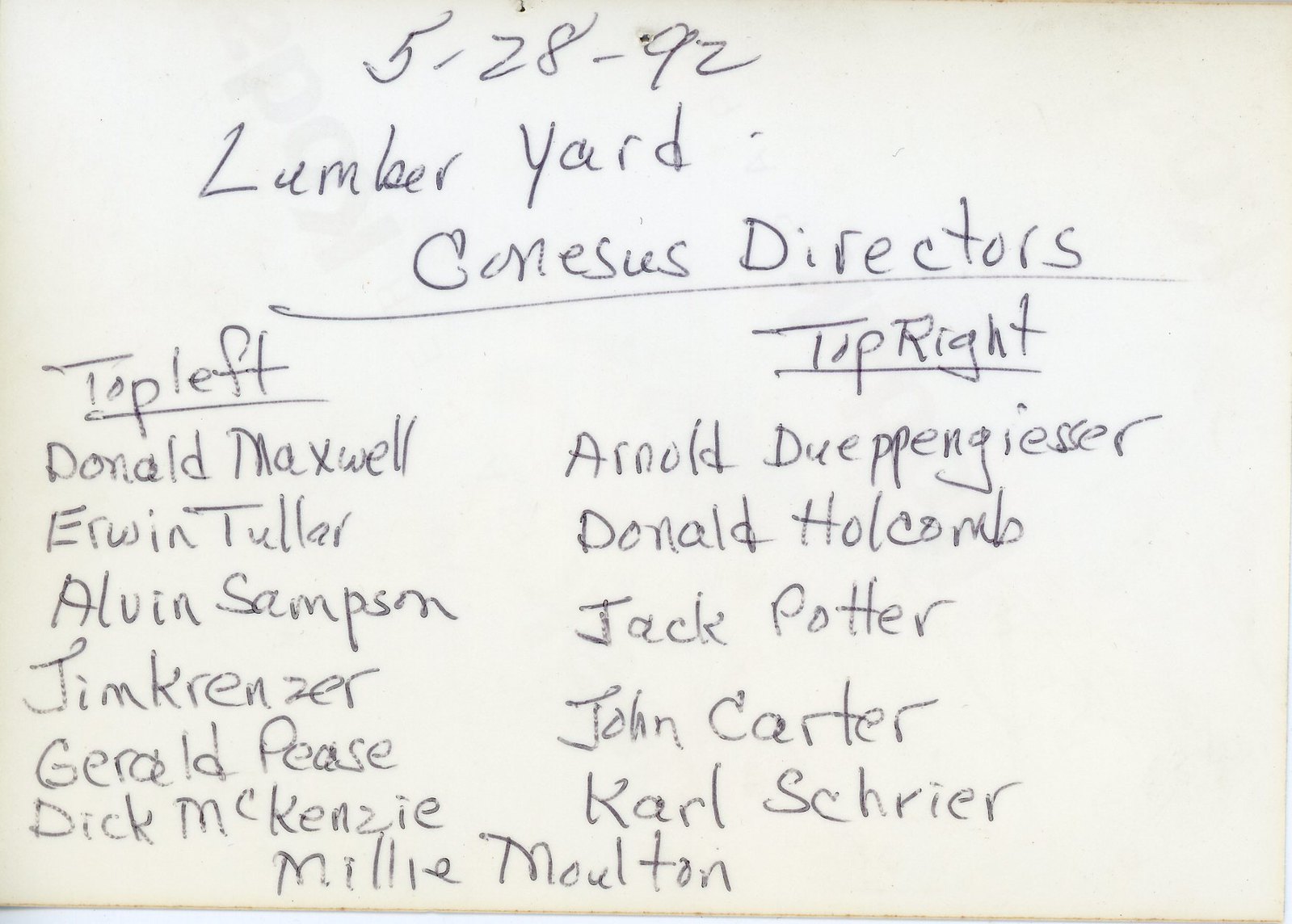The image is a detailed, handwritten note on a piece of paper dated 5-28-92. It features the word "Lumberyard" prominently in the top middle. Directly below "Lumberyard" and starting from the 'R' is the underlined heading "CONESUS Directors." This is followed by two separate sections divided into "TOP LEFT" and "TOP RIGHT," each heading underlined.

Under "TOP LEFT," there is a list of six names:
1. Donald Maxwell
2. Erwin Tuller
3. Alvin Sampson
4. Jim Krenzer
5. Gerald Pease
6. Dick McKenzie

Under "TOP RIGHT," there is a list of five names:
1. Otto Dwebbingeser
2. Donald Holcomb
3. Jack Potter
4. John Carter
5. Carl Schroer

At the bottom of the paper, the name "Millie Moulton" is written, spanning from the left section to the right section. The note does not include any logos or additional indications about the nature of "Lumberyard," and it remains uncertain whether "CONESUS Directors" refers to a company board or a city council. The entire note is handwritten, with no additional context provided about the entity named "Cadizes," which remains ambiguous.